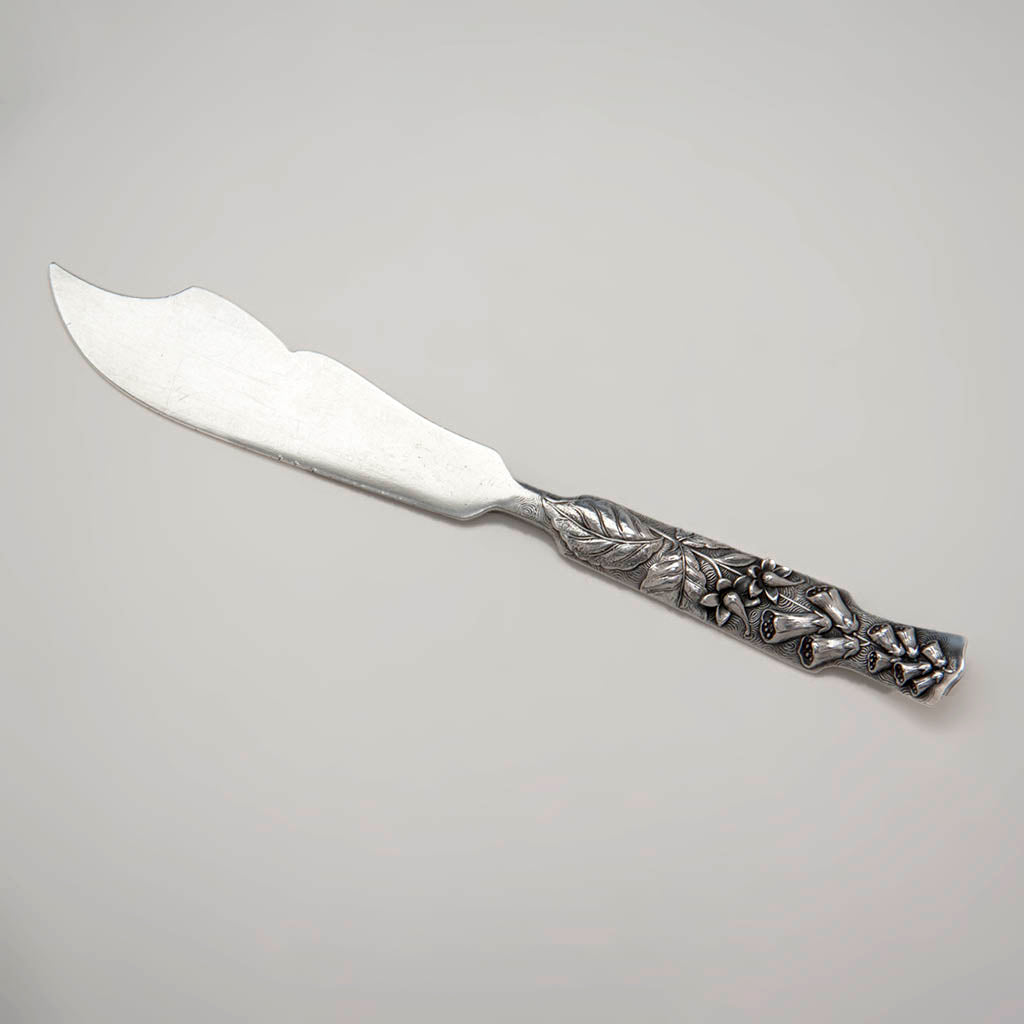This image depicts a silver knife elegantly placed against a simple gray background. The background itself is subtly shaded, getting darker at the corners. The knife, likely made of real silver, features an intricately embossed handle. This handle showcases a detailed design of leaves, stems, and bell-shaped flowers, resembling a winter berries and bells scene. The blade of the knife is quite unique, with a shape reminiscent of a scimitar; it curves downward at the bottom and has at least three grooves along the top, leading to a pointed tip on the left side. Positioned diagonally, the handle appears closer to the bottom right of the image, while the blade extends towards the top left. The ornate nature of the knife, particularly the handle, suggests it could be part of an exquisite silver serving set, likely used as a cheese knife.